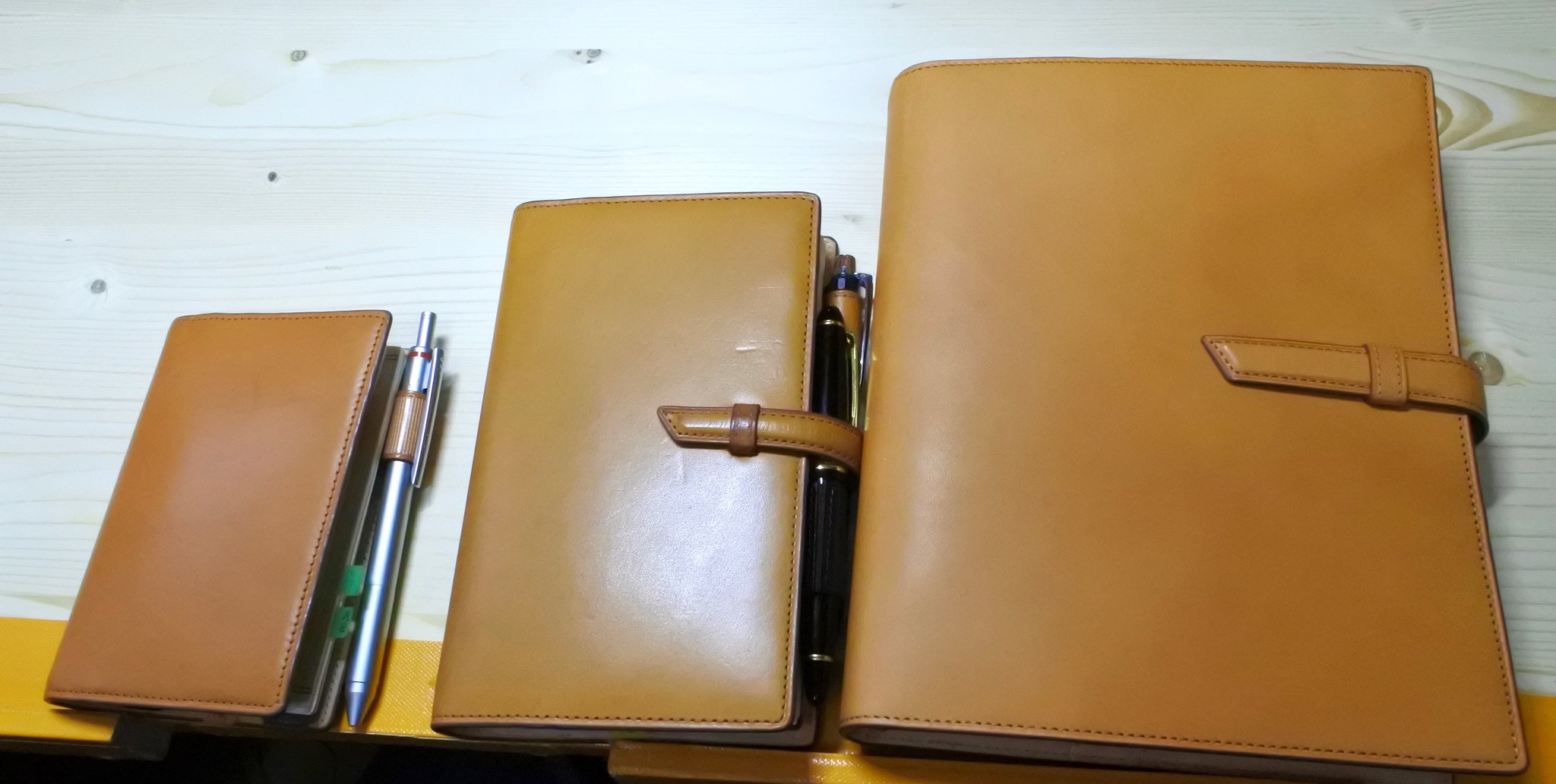The image showcases three medium brown leather cases of varying sizes arranged on an off-white wood background with orange trim at the bottom. The smallest case, likely a checkbook holder, features a silver pen with a blue end nestled in its pen holder. The medium-sized case appears to be a wallet, characterized by its layers and central clasp for closure. The largest case resembles a legal pad folder, and similarly to the others, has a central clasp for closure. All three items boast a cohesive design with a leather-like finish, enhancing their elegant and functional appearance.